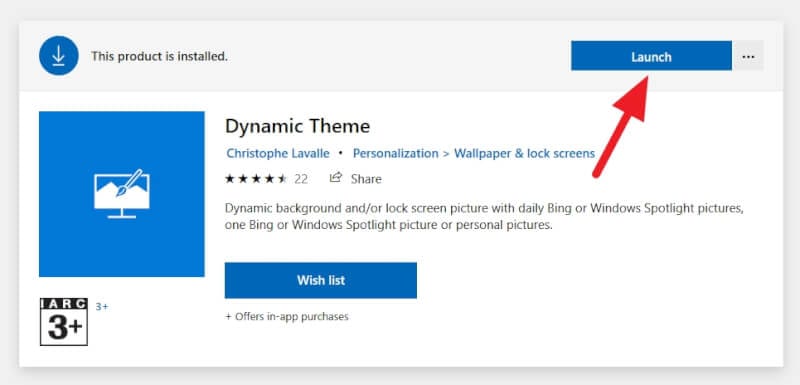This is a detailed description of a screenshot from an app. On the left-hand side, there is a blue download button with an arrow and the text "This product is installed." On the right-hand side, there is a rectangular blue button labeled "Launch" with a large red arrow pointing to it.

In the main part of the image, there is a large blue box on the left containing a computer icon and a paintbrush on the computer screen. The title "Dynamic Theme" is displayed in black text, followed by the name "Christopher Lavelle" in blue. Additional details include the categories "Personalization", "Wallpaper and Lock Screens", a rating of four and a half stars, and the number "22". Directly below these details is a share icon accompanied by the word "Share".

Further down, there is a description that reads: "Dynamic background and/or lock screen picture with daily Bing or Windows Spotlight pictures, one Bing or Windows Spotlight picture or personal pictures." Beneath this, there is another blue rectangular button labeled "Wishlist," followed by a note in small black text stating "Offers in-app purchases."

In the bottom left corner of the screenshot, there is a small black and white box labeled "IARC" with "3+" inside it and a smaller "3+" outside the box.